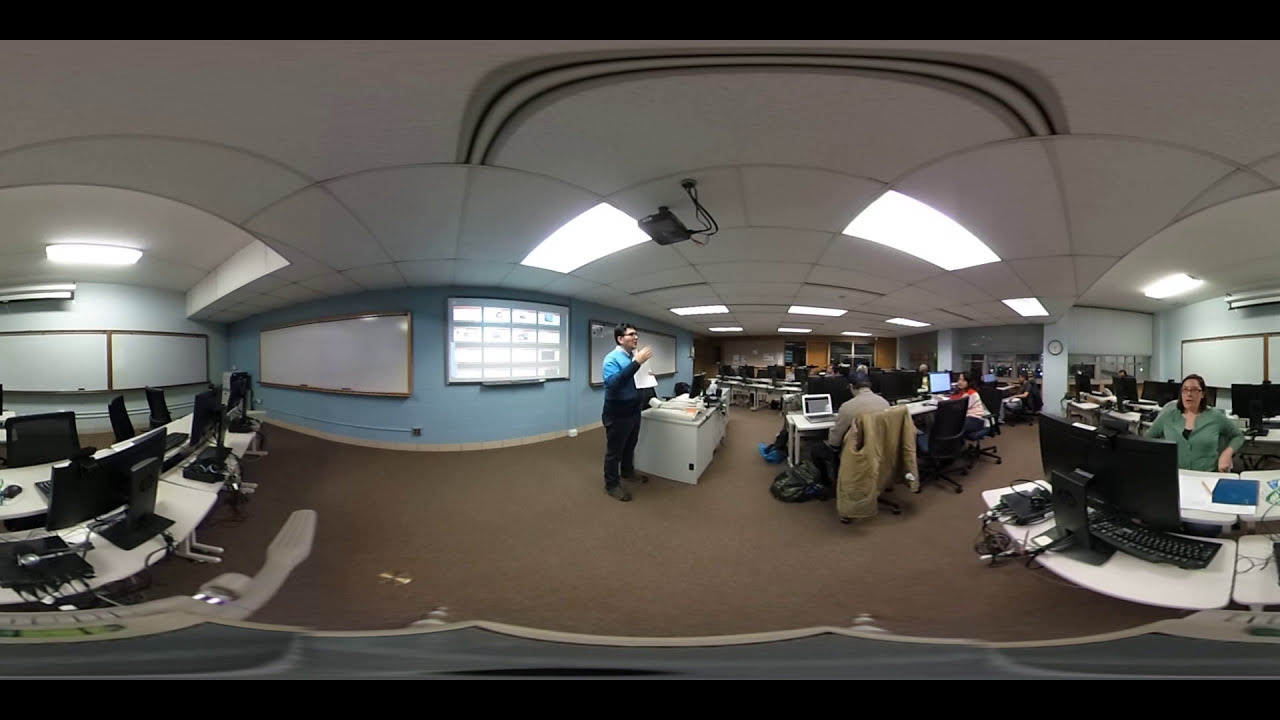The photograph captures a slightly distorted, wide-angle view of a spacious office environment with blue walls and a boring brown carpet. The image shows a series of white desks equipped with black computer monitors and assorted office chairs, all arranged throughout the room. Fluorescent lights line the slightly curved ceiling, which also holds a slide projector.

In the center of the image, a man is standing next to a desk. He's donned in dark pants, brown shoes, a blue shirt, and eyeglasses, holding a piece of paper as if he's giving a presentation or speaking to the room. To his right and scattered throughout the room, various workers are seated at computers. Notable among them are a man in a brown coat and a woman in a green blouse, both engrossed in their work. Despite the abundance of computer workstations, the room is only sparsely populated, with around a dozen individuals present. Whiteboards are interspersed all around, on the walls to the left, right, and even behind the standing man, indicating a versatile workspace designed for both individual work and collaborative activities.